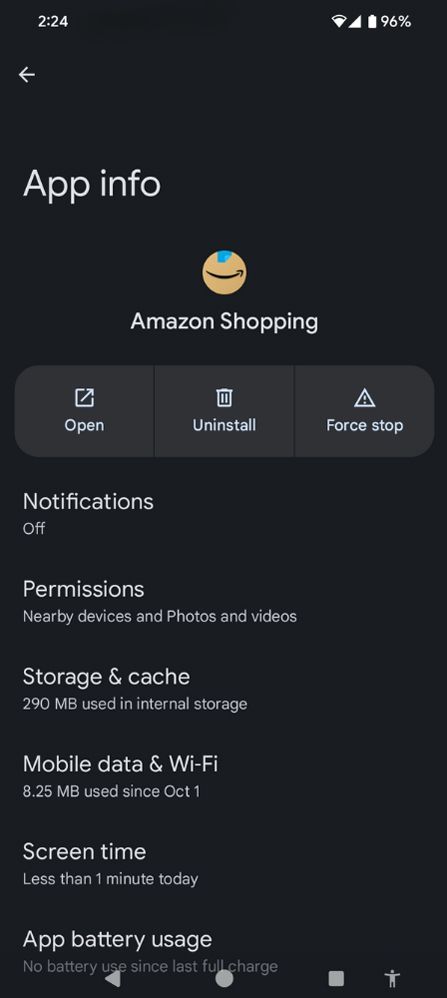This image captures the details of a smartphone screen displaying the app information for Amazon Shopping. The background is entirely black, which highlights the interface elements. At the very top of the screen, the time is shown as 2:24, with the battery charge visible at 96%, along with icons for Wi-Fi connectivity and a triangular symbol. The most prominent text, "App info," is displayed at the top.

Beneath that, the app name "Amazon Shopping" is written in white text, accompanied by its icon—an image resembling a cardboard box within a circle, featuring the recognizable Amazon swoosh logo. Three actionable buttons are clearly visible: "Open," "Uninstall," and "Force stop."

Further down, the interface indicates that notifications are turned off. The permissions section lists access to nearby devices and photos and videos. Below that, the storage and cache information reveals that the app uses 290 MB of internal storage. Additional details include sections for mobile data and Wi-Fi, screen time, and app battery usage at the very bottom of the screen.